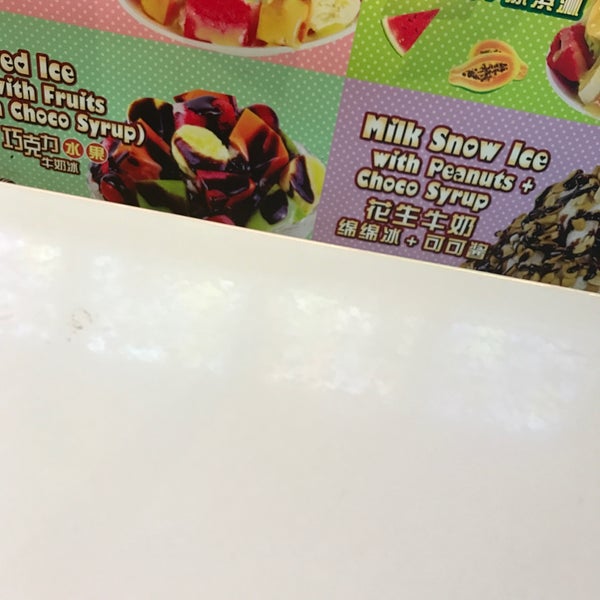The image captures a colorful advertisement sign, likely for a dessert shop or a healthier alternative dessert store. Dominating the upper portion of the image is a segmented menu featuring vibrant colored sections: the top left is pink, the top right is lime green, the bottom left is a mint green color, and the bottom right is purple with white polka dots. The colorful sections feature various dessert offerings and text in both English and Chinese. 

The visible menu items include "Milk Snow Ice with Peanuts plus Choco Syrup" and "Mixed Ice with Fruits and Choco Syrup". Each description is accompanied by appealing photographs of the desserts, such as bowls of fruit drizzled with chocolate syrup. The white surface below these colorful segments reflects some light and occupies the bottom half of the image, creating a distinct separation between the advertisement and the background. The objects in the advertisement, including peanuts, chocolate syrup, watermelon, and other fruits, are strategically positioned towards the top, making them the focal point. The overall setting suggests it might be a restaurant menu or a sign on a vending machine, aimed at enticing customers with its vibrant and appetizing visuals.